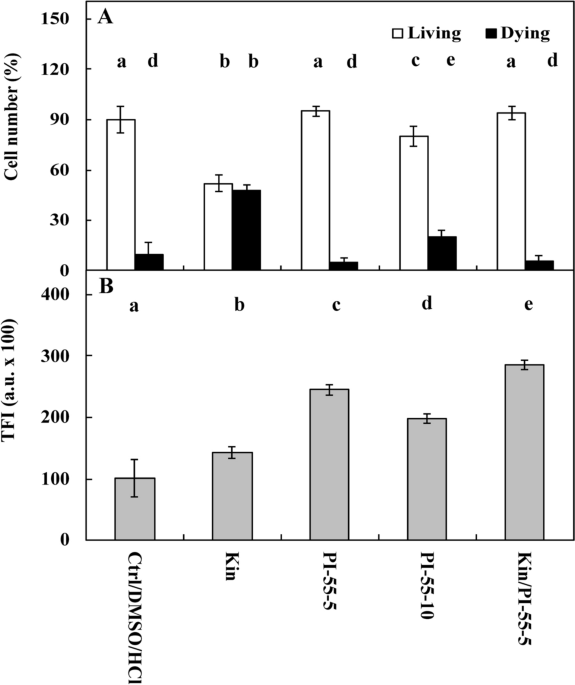This image presents a detailed comparison through two bar graphs. The upper graph displays five sets of vertical bars labeled A, B, C, D, and E. Each set contains a white bar indicating 'living' and a black bar indicating 'dying.' The vertical axis of the top graph measures cell numbers in terms of percent, ranging from 0 to 150. There is a key in the upper right corner that clearly differentiates between the white and black bars.

The bottom graph features gray bars, also in five sets, each representing different experimental conditions. These are labeled with combinations of letters and numbers: CTRL/DMSO/HCL, KIN, PI-55-5, PI-55-10, and KIN/PI-55-5. The vertical axis for this graph measures TFI (in AU times 100) from 0 to 400. Each bar in the bottom graph has a line through it, possibly indicating a range of measures, with the bar itself showing the average.